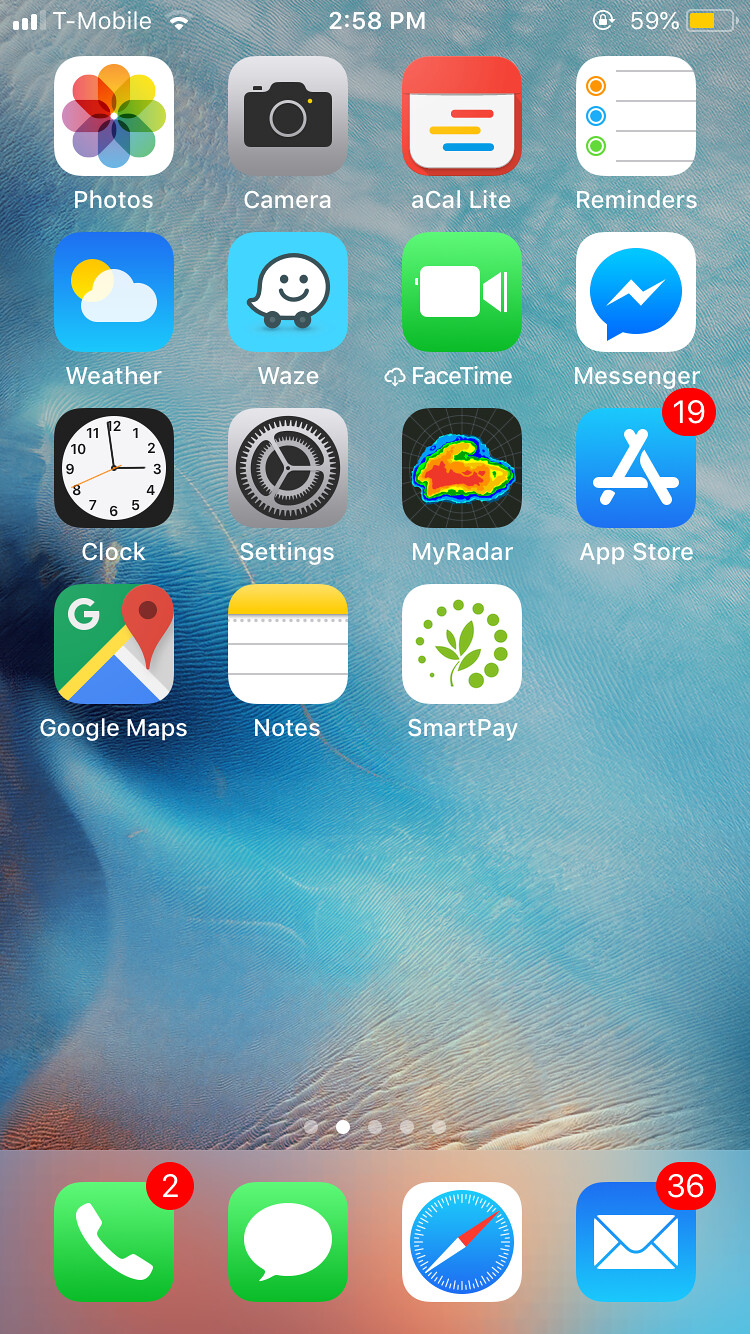The image displays the home screen of a mobile phone. In the status bar at the top, "T-Mobile" is indicated as the service provider, showing strong signals for both Wi-Fi and cellular networks. The current time is 2:58 p.m., and the battery is at 59%, represented by a yellow battery icon that is more than half full.

The home screen is populated with various apps. Notable ones include:

- **Photos**: An app represented by a rainbow-colored flower icon.
- **Camera**: Illustrated by a camera icon.
- **A-Cal Lite**: A red app icon featuring blue, yellow, and red lines.
- **Reminders**: Depicted with an icon showing lines.
- **Messenger**: Sporting the Facebook Messenger logo.
- **MyRadar**: Represented by an icon similar to a radar scan typically seen in weather stations.
- **Notes**: With an icon of a white page featuring lines and a yellow top.
- **Google Maps**: Showing the usual map pointer icon.
- **Clock**: Displaying a classic clock face with the time set to two minutes before 3 o'clock, complete with a sweeping second hand.
- **Waze**: A light blue icon with a smiley, cartoonish white face.
- **FaceTime**: Featuring the recognizable green video camera icon.
- **SmartPay**: The icon for this app is also visible.

All icons are neatly arranged, providing quick access to these various applications.